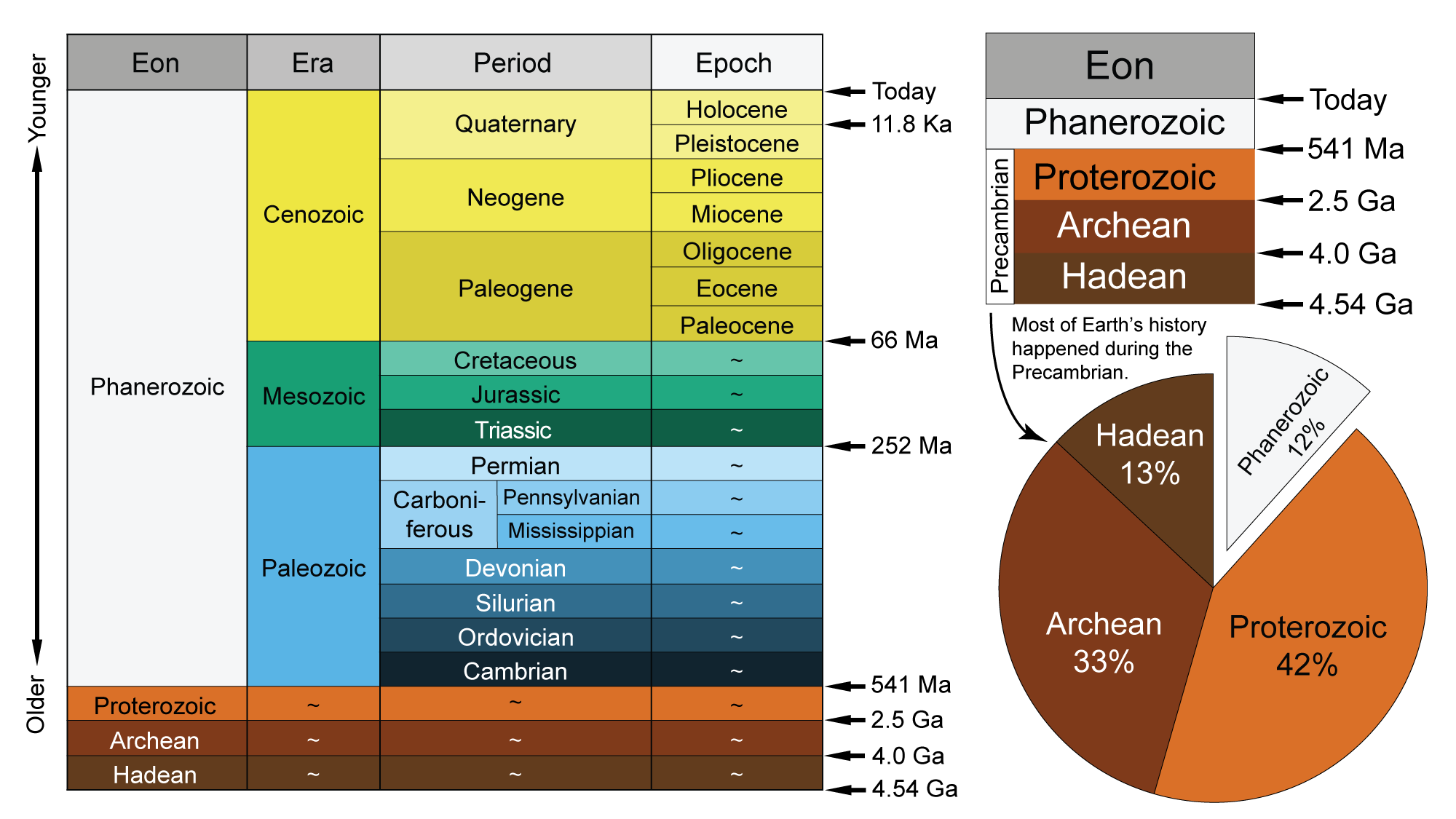This image depicts a detailed chronological table and pie chart that organizes Earth's history into Eons, Eras, Periods, and Epochs, labelled at the top. The main graphic, a large multicolored table, is divided into different hues of yellow, green, blue, and brown, representing various segments of geologic time. Vertically on the left, it is ordered from older to younger epochs and periods, including the Phanerozoic Eon, Cenozoic Era, Mesozoic Era, Paleozoic Era, Proterozoic Eon, Archean Eon, and Hadean Eon, with detailed subdivisions such as the Quaternary, Neogene, and Paleogene Periods, among others. On the far right, an additional vertical table with an orange color spectrum delves into more specific subdivisions. Below this, a pie chart provides a segmented view with sections in white, orange, reddish brown, and brown, emphasizing that most of Earth's history occurred during the Precambrian time.